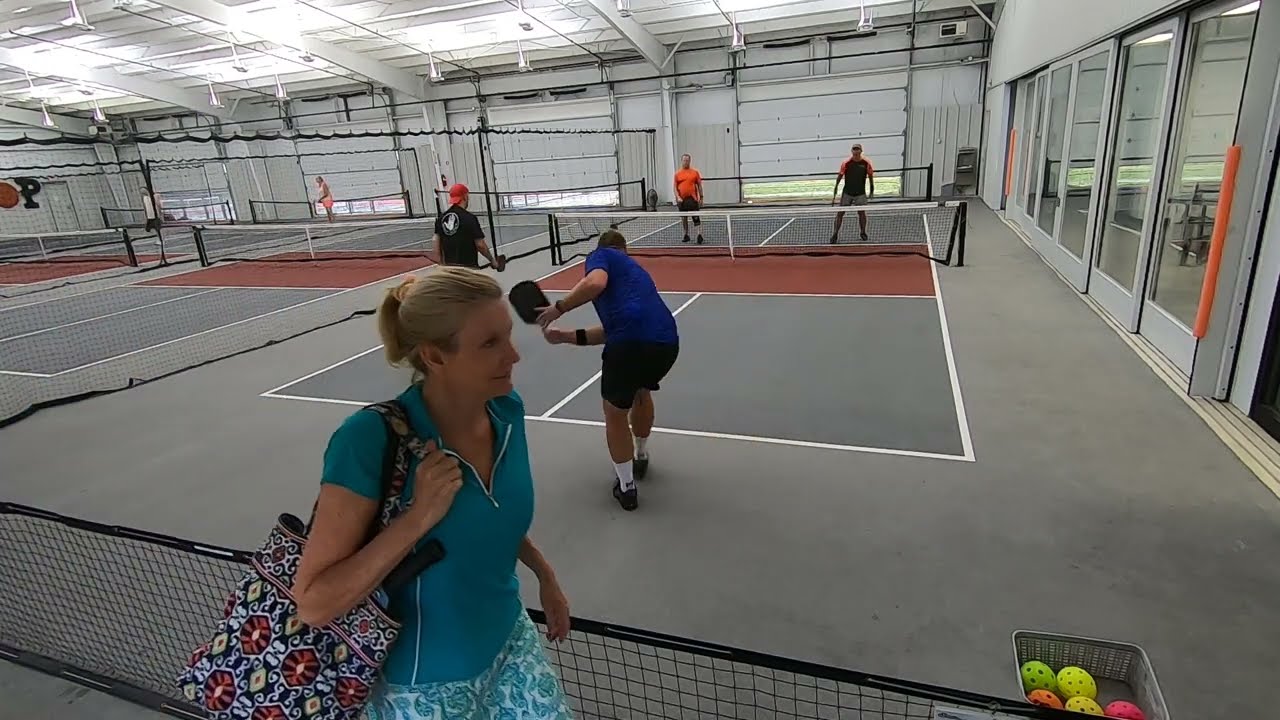In an expansive indoor facility resembling a white-walled gymnasium or warehouse with partially open garage doors for ventilation, a scene unfolds of bustling pickleball activity. There are three pickleball courts visible, all actively being used. Dominating the foreground, a Caucasian woman with blonde hair in a ponytail wears a turquoise blue short-sleeved shirt and a blue skirt. She carries a flowery bag on her right shoulder as she walks past a low waist-high net, seemingly designed to keep pickleballs from rolling off the court.

Behind her, a doubles match is in progress on the nearest court, with four male players fully engaged in the game. One man, sporting a blue shirt, appears poised to either start or return a serve, while his three opponents are positioned at the ready. The court to the left of the match also hosts players, indicating all courts are occupied. To the far right, situated by some glass windows and a metal wall, is a basket containing a variety of pickleballs—some yellow and orange, others green and pink, all marked with holes quintessential to the sport. The overall ambiance is brightly lit, capturing the energetic pulse of a pickleball day within this multi-functional space.